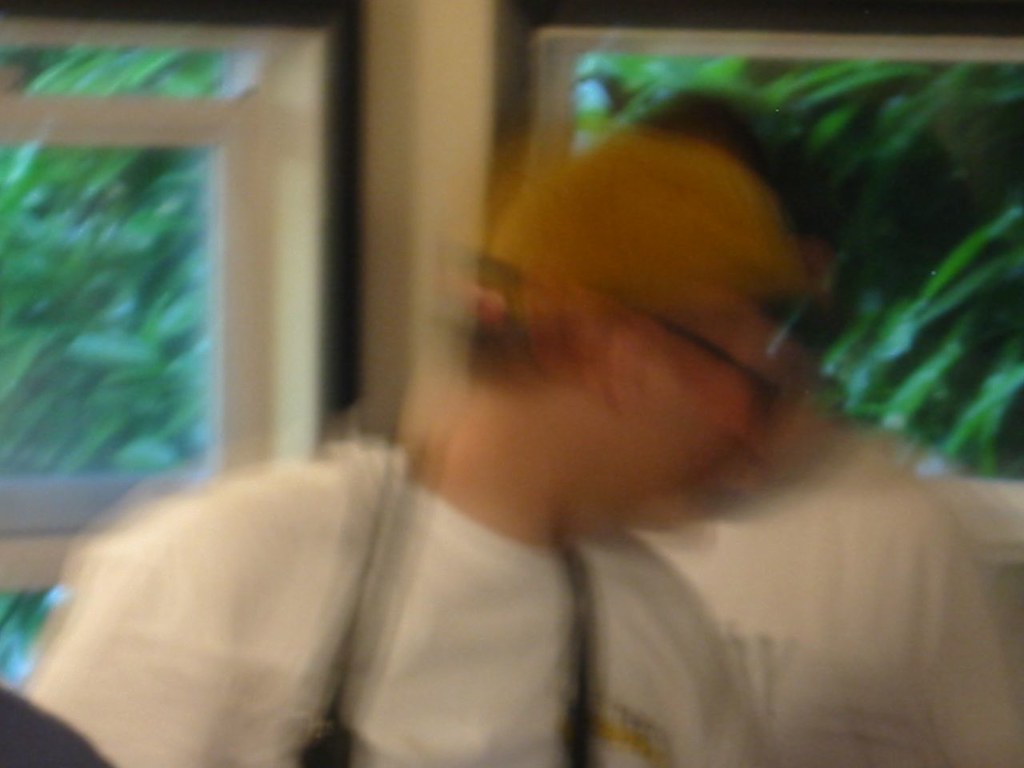In this image, the scene is set indoors with large windows in the background that have white frames. Through these windows, a lush expanse of greenery is visible, suggesting an outdoor area rich with foliage. The lighting suggests it is near dusk, as it appears darker than light outside. In the foreground, there are two figures who are both very blurry. The person in front is wearing a yellow cap, glasses, and a white t-shirt, with what seems to be binoculars hanging around their neck. The second person, positioned behind the first, is also wearing a white t-shirt and either a black cap or has dark hair. Their face is obscured by the person in front. The exact location remains unidentified.